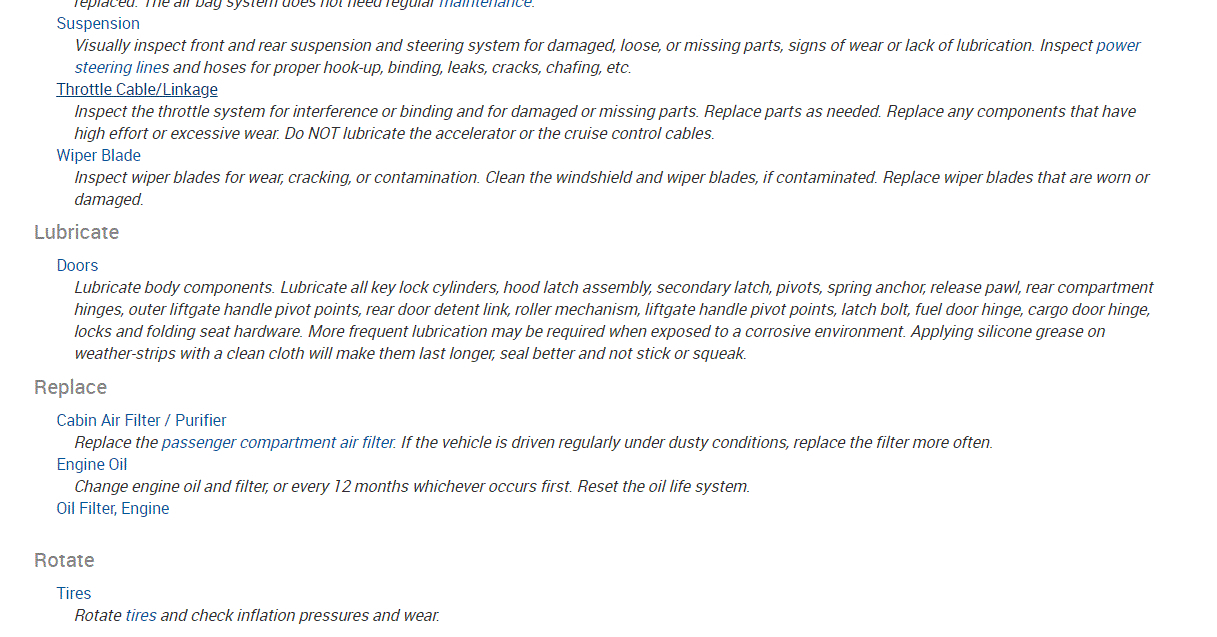The image contains detailed instructions related to the maintenance and inspection tasks for a vehicle. The text is structured into several sections addressing different components and systems of the vehicle.

1. **Bag System**: The text indicates that the bag system has been replaced and does not require regular maintenance.

2. **Suspension**: 
    - **Visual Inspection**: Conduct a thorough visual inspection of both the front and rear suspension and steering systems.
    - **Components Check**: Look for any damaged, loose, or missing parts, indications of wear, and any lack of lubrication.
    - **Power Steering**: Inspect the power steering lines and hoses for proper binding, leaks, cracks, or signs of chafing.

3. **Throttle Cable Linkage**:
    - **Inspection**: Examine the throttle system to ensure there is no interference, binding, damage, or missing parts.
    - **Component Replacement**: Replace any components showing high effort or excessive wear. It is essential not to lubricate the accelerator or the cruise control cables.

4. **Wiper Blades**:
    - **Inspection**: Check for wear, cracking, or contamination on the wiper blades.
    - **Cleaning**: Clean both the windshield and the wiper blades if contamination is present.
    - **Replacement**: Replace any wiper blades that are worn or damaged.

5. **Lubrication**:
    - **Doors**: This section appears to provide instructions on lubricating the vehicle's doors, though further details are not included in the excerpt.

6. **Replacement**: This section likely details various components that need periodic replacement, though specific items are not listed in the given text.

This image guide serves as a comprehensive checklist for ensuring the vehicle's components are in optimal condition through regular inspection and maintenance.